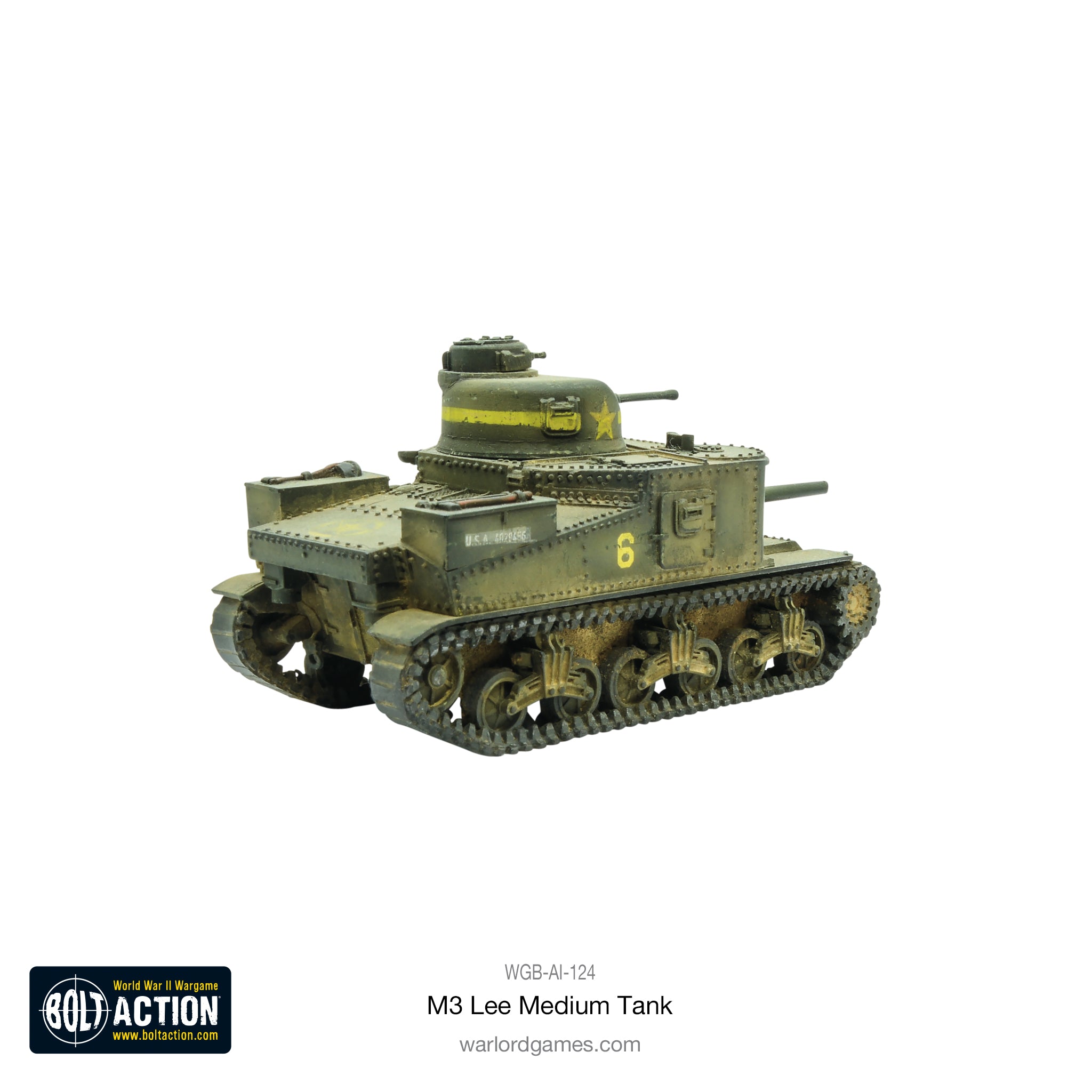This detailed photograph portrays a miniature model of an M3 Lee Medium Tank, primarily used in a World War II war game labeled as "Bolt Action" from warlordgames.com. The tank, painted in army green with a greenish-yellow hue, features distinct design elements such as tank treads with black tracks and circular gears. Prominently, it displays a yellow stripe encircling the turret and a yellow star atop the hatch area. The side of the tank is marked with the number 6 in yellow, and additional markings include "USA" in white print. The model incorporates multiple guns: one extending from the front hull, another from a smaller turret atop the main body, and potentially a third from another elevated turret position. Labeled beneath the image is the identifier "WGB-AI-124 M3 Lee Medium Tank" with the website warlordgames.com, providing further context and authenticity to the model.